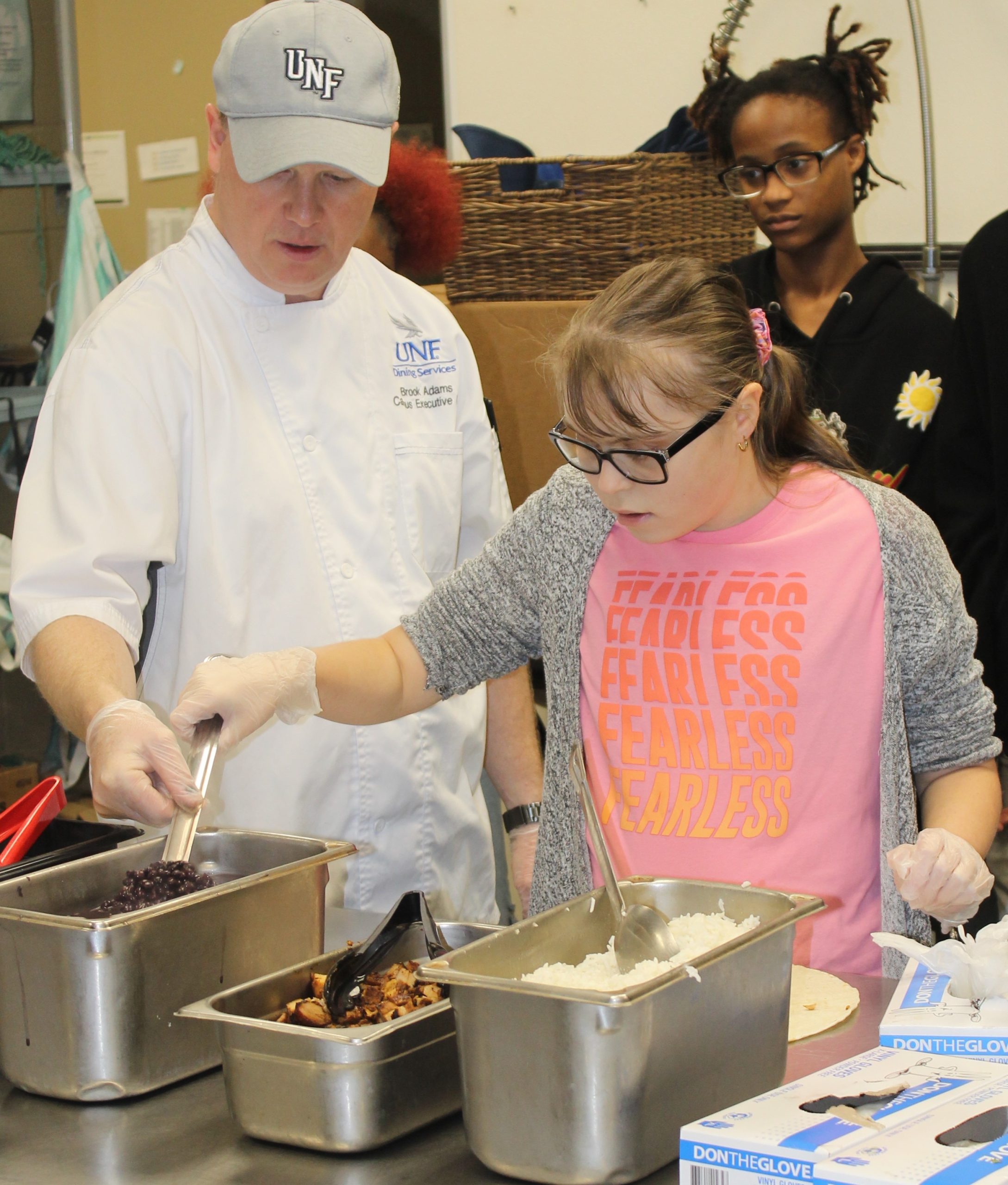In this detailed photo, a chef named Brooke Adams is guiding a young Caucasian girl with Down syndrome, in a white kitchen attire emblazoned with "UNF." Brooke, who wears a gray UNF cap and short-sleeved chef's coat, stands on the left, glowing with professionalism. The girl beside him is dressed in a pink and orange "fearless" t-shirt under a gray sweater, accessorized with black-rimmed glasses and a pink bow in her brown hair. Both are equipped with white latex gloves, and together they stir black beans in a large oval-shaped silver bowl. On the shiny stainless steel countertop before them are three rectangular stainless steel bins common in restaurant settings, holding black beans, fried potatoes, and rice. In the background, figures in black jerseys with insignias move about, and a wicker basket and cardboard boxes rest on the surfaces. A young black girl in a smock with yellow flowers and braided pigtails observes the cooking, adding to the scene's lively ambiance.